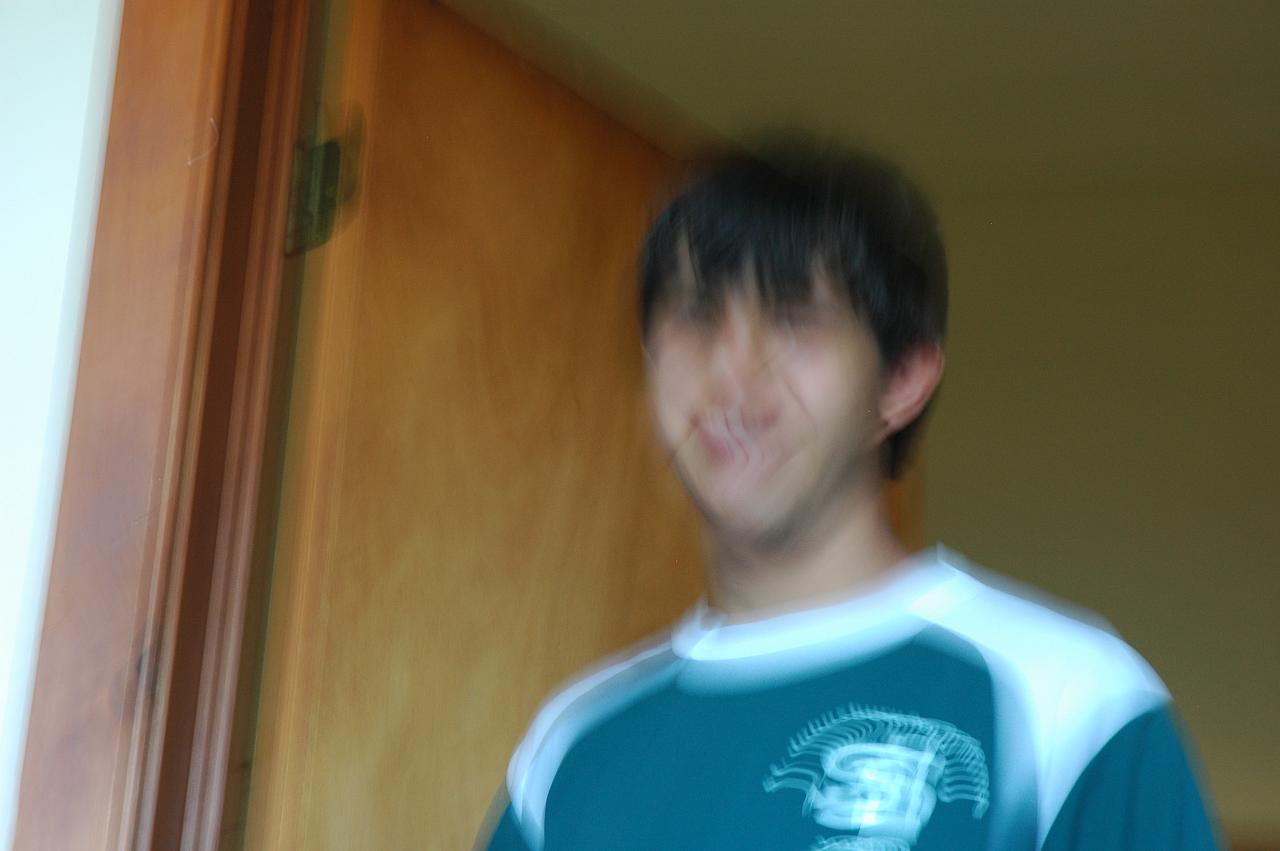A blurry image captures a teenage boy standing in the doorway of an open, light brown door with metal hinges on the left. He has dark hair styled with bangs that fall into his eyes, which are dark and possibly smiling. His face is slightly distorted due to the motion blur or double exposure. He wears a blue and white t-shirt featuring an S-shaped logo with lines extending from it, reminiscent of a soccer jersey. The door frame's molding is dark brown, contrasting with the white wall outside the doorway. Despite the blur, the boy’s light skin and cheerful expression are discernible, suggesting he might be Caucasian or Asian.